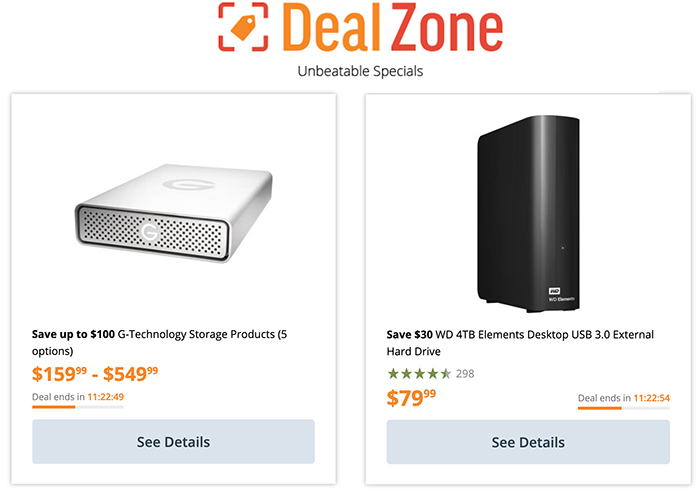At the top and center of the image, there is a "Deal Zone" label. The word "deal" is in orange, and the word "zone" is in red. The label is enclosed in a square bracket design, with orange brackets at the top-right and bottom-left corners, and red brackets at the top-left and bottom-right corners. In the center of the square is an orange tag icon.

Below the "Deal Zone" label, the phrase "Unbeatable Specials" is prominently displayed.

The image features two highlighted deals, each within a vertically oriented rectangle with a gray border.

**Left Rectangle:**
- **Title:** "Save up to $100 on G-Technology Storage Products"
- **Description:** Features five different hard drive options.
- **Price Range:** $159.99 to $549.99
- **Countdown Timer:** Deal ends in 11 hours, 22 minutes, and 49 seconds.
- **Status Bar:** Displayed as half orange and half gray, indicating deal progress.
- **Details Button:** Gray button labeled "Details"

**Right Rectangle:**
- **Title:** "Save $30 - WD 4TB Elements Desktop USB 3.0 External Hard Drive"
- **Visual:** Image of the external hard drive standing upright.
- **Rating:** 4.5 stars, based on 298 reviews.
- **Price:** $79.99
- **Countdown Timer:** Deal ends in 11 hours, 22 minutes, and 54 seconds.
- **Status Bar:** Displayed as half orange and half gray, indicating deal progress.
- **Details Button:** Gray button labeled "Details"

Both rectangles are surrounded by a thin gray outline, neatly framing the information.